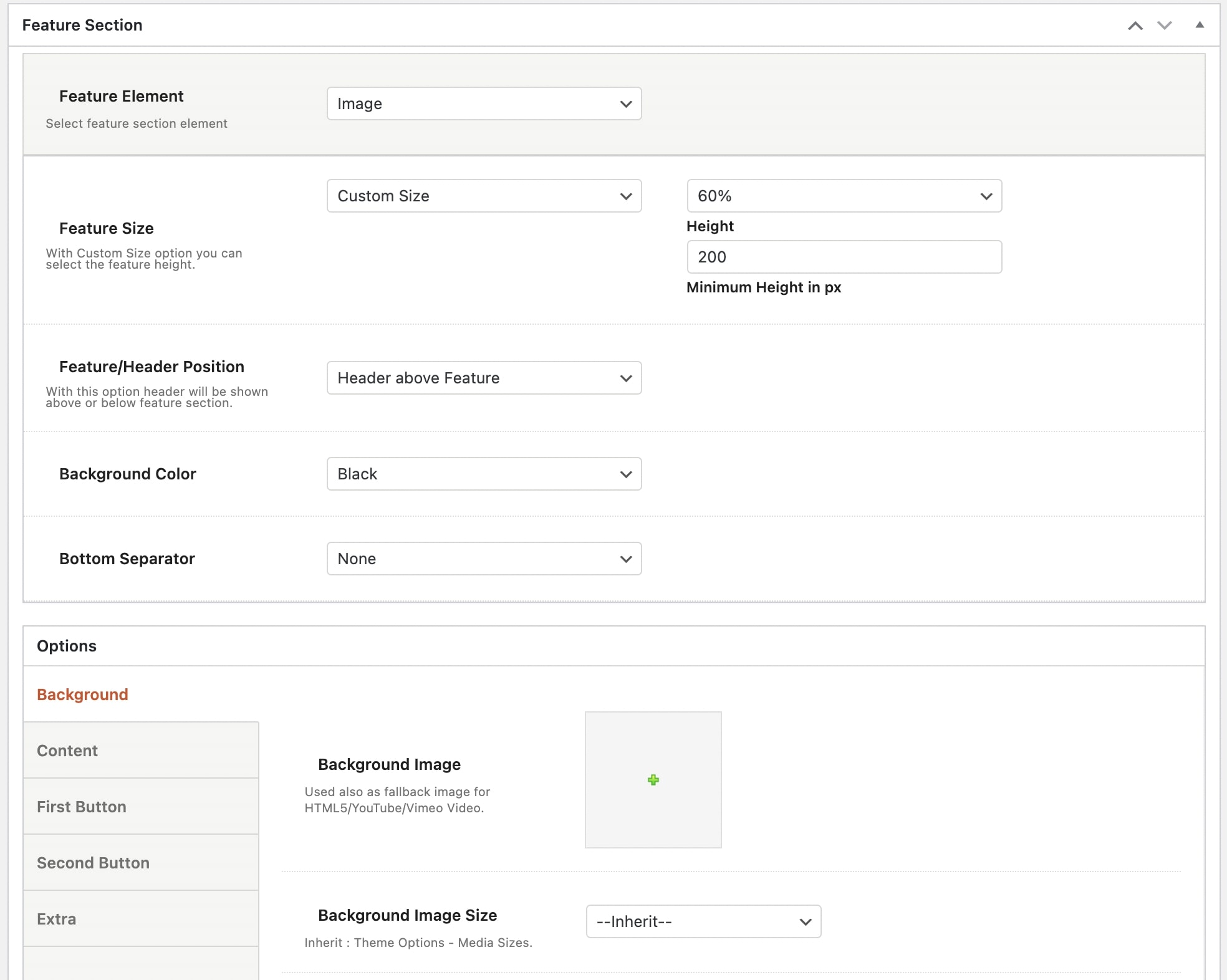This screenshot depicts an application interface featuring various customizable settings. 

At the upper left, there's a section labeled "Feature Section," flanked by an up arrow, a down arrow, and another up arrow on the right side. Below this, the bolded header "Feature Elements" prompts users to "Select Feature Section Element," with a dropdown menu next to it showing "Image" as the chosen option.

The next section is labeled "Feature Size," and includes a subtitle: "With custom size option, you can select the feature height." To the right is an option for "Custom Size," currently set at 60% height. Directly beneath this is a "Minimum Height in PX" field set to 200.

Following this is the "Feature Header Position" section, explaining that users can choose whether the header appears above or below the feature section. Presently, "Header Above Feature" is selected.

Next is the "Background Color" section, with black chosen as the current color. Below that, the "Bottom Separator" section shows that none is selected.

Further down, there's a section labeled "Options" for the background, featuring multiple selections like "Content," "First Button," "Second Button," and "Extra," with "Background" highlighted in orange. Under the "Background" option, users can set a "Background Image" and also choose a fallback image for HTML5/YouTube/Vimeo videos. Adjacent to this is a gray square with a green cross in the center.

Lastly, the "Background Image Size" section indicates the current setting to "Inherit Theme Option Media Sizes," with "Inherit" selected.